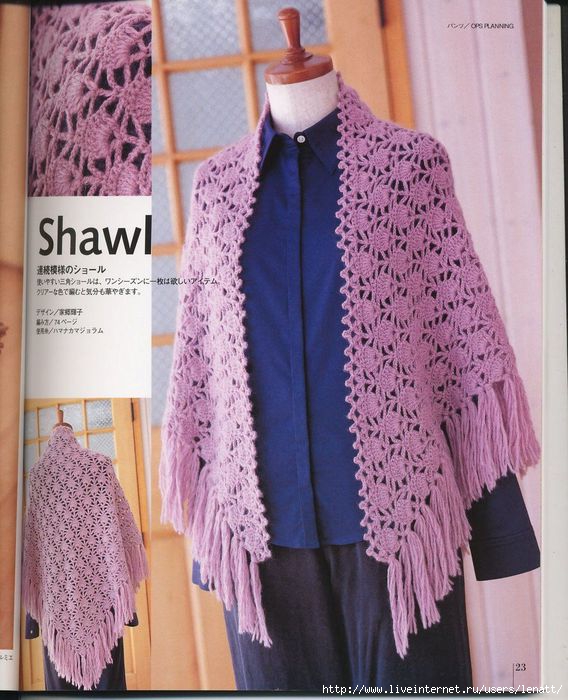The image features a headless, armless mannequin dressed in a beautifully crocheted shawl, positioned in front of a wooden door. The mannequin is outfitted with gray pants and a navy blue button-up shirt. The focal point is a delicate lavender shawl, adorned with an intricate floral pattern and finished with fringe all around its edges. The shawl elegantly drapes over the mannequin’s shoulders, showcasing its length and design, particularly noticeable in the lower left corner where the back view of the shawl is highlighted. Additionally, the top left corner offers a close-up view, detailing the complexity of the floral crochet work. The image appears to be styled as a magazine page, with the word "shawl" boldly printed on the left, accompanied by some text in Chinese or Japanese characters beneath it.